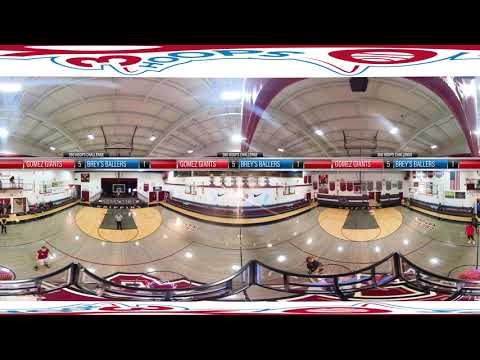This image is a distorted panoramic view of a basketball court, capturing two spliced halves that create a fisheye effect. The court floor appears predominantly gray with an area of natural wood color, and the surroundings include white walls and a visible white ceiling with metal roof supports. Included in the scene are several people: a referee stands at center court on the left side, accompanied by a few spectators in the bottom left corner, while on the right side, multiple people are milling about in various positions. A ticker tape banner stretches across the middle and top of the image, displaying the teams' names and scores: it reads "Gomez Giants 5, Gray's Ballers 1" across the middle and "3 Hoops" at the top, although the text is slightly distorted. The entire image is framed by thick black rectangles at the top and bottom, giving it a bordered effect. The panorama effect creates the illusion of two almost identical halves, contributing to the unusual visual distortion of the scene.